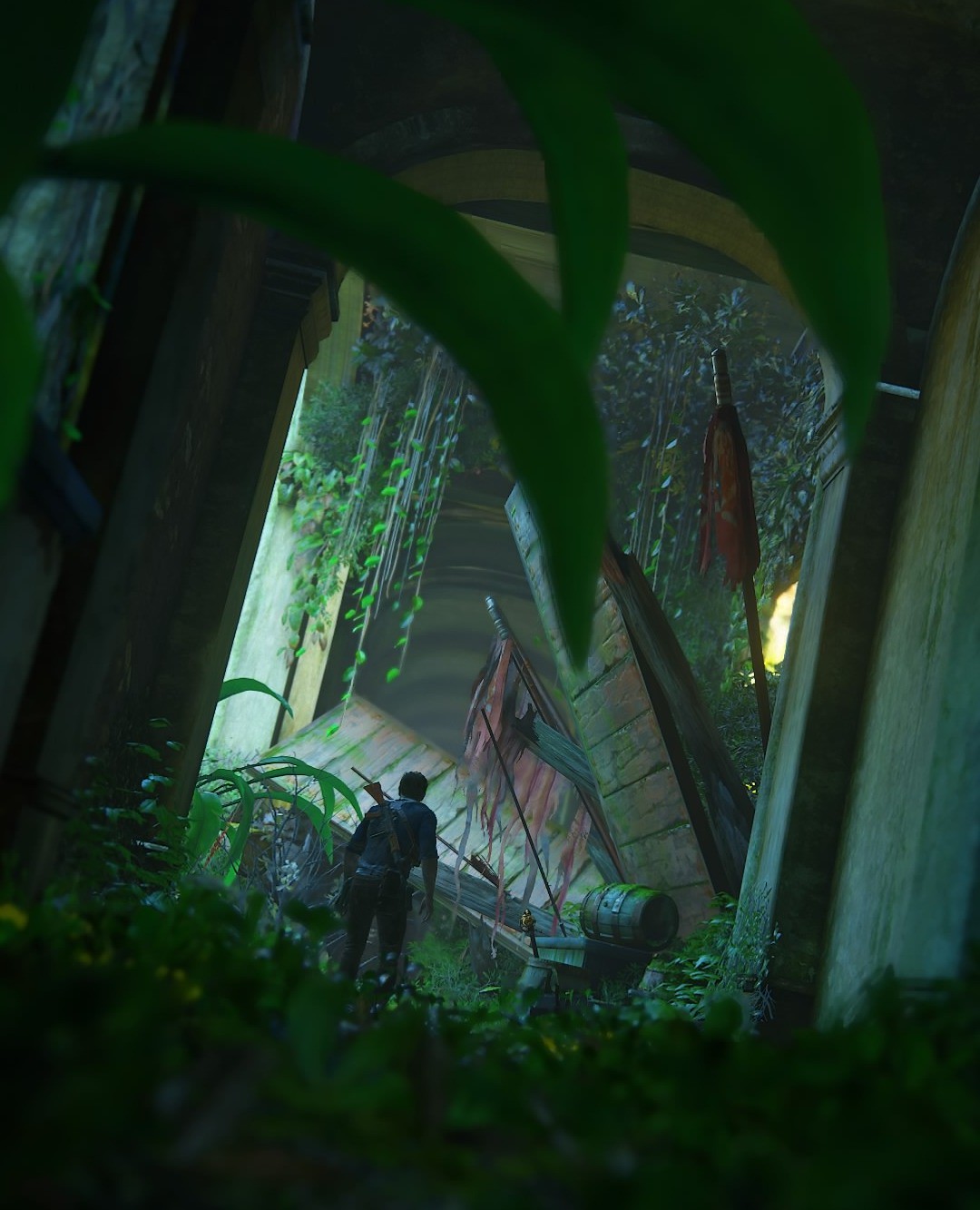In this detailed still from an animated video game or movie, we peer through layers of lush vegetation. At the top of the frame, long, curved green leaves cascade downward, partially obscuring the view. The lower part of the scene is filled with dark and light green foliage, creating a dense and vibrant foreground. 

Beyond this verdant frame, the focus shifts to a lone figure dressed entirely in black, who is seen walking away from the viewer. The character is making their way through an ancient, deteriorating archway that likely leads to long-forgotten ruins. The portal they pass through hints at a rich history, evidenced by the tattered, ragged flag fluttering nearby. Surrounding the archway, time-worn wooden panels lean precariously, and a barrel lies on its side, adding to the scene's air of abandonment and decay.